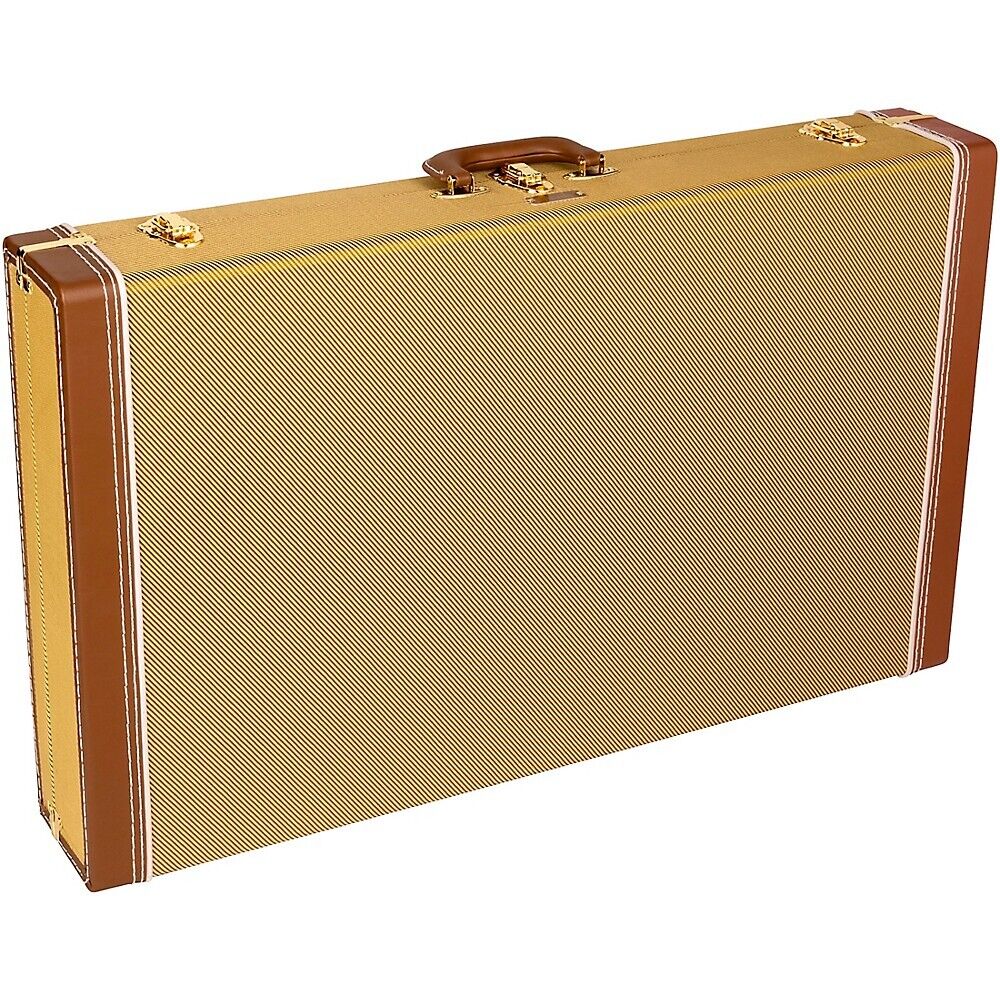This photograph features a sleek, slim briefcase set against a completely solid, opaque white background, suggesting that the image has been carefully edited to remove any distractions. The briefcase is positioned upright and slightly angled away from the viewer, highlighting its elegant design. 

The briefcase boasts a sophisticated beige-tan color scheme, with a warm yellowish-brown handle of medium depth that coordinates with the trim along the edges. The hardware, consisting of three locks along the top, is a striking gold or brass color, adding a touch of luxury to the utilitarian piece. 

The primary fabric of the briefcase features a subtle pattern of diagonal lines, alternating between a very light yellowy-beige and black. This intricate design blends to create an overall impression of a refined yellowy-beige hue, complementing the briefcase's understated yet classy aesthetic.